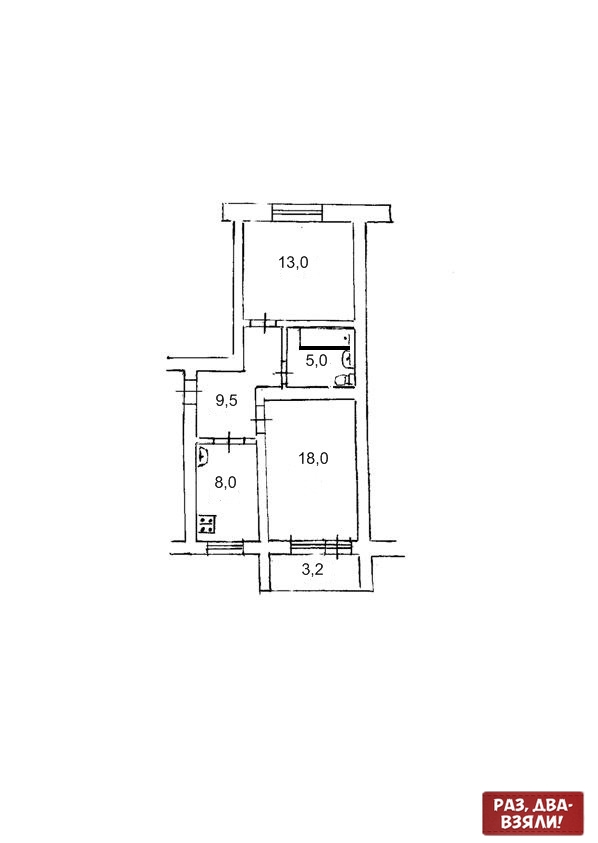This image depicts a detailed architectural blueprint of a house layout featuring five primary rooms with specified measurements. Starting from the left, the front room measures 13-0 and includes a door that opens into a larger room measuring 19-5. Adjacent to this room is a bathroom, measuring 5-0, which includes a toilet, sink, and bathtub. Additionally, there's a hallway labeled 9-5 next to the bathroom. Moving towards the larger section, there's a significant room marked 18-0, which leads into a smaller room labeled 8-0. Below this large room, there's a small closet-like space measuring 3-2. The entire layout is annotated with coordinates, and in the bottom right corner, a red text box features the text "PA3, ABA-B3RAN." The blueprint appears in a primarily white space, indicating unutilized areas around the planned rooms.